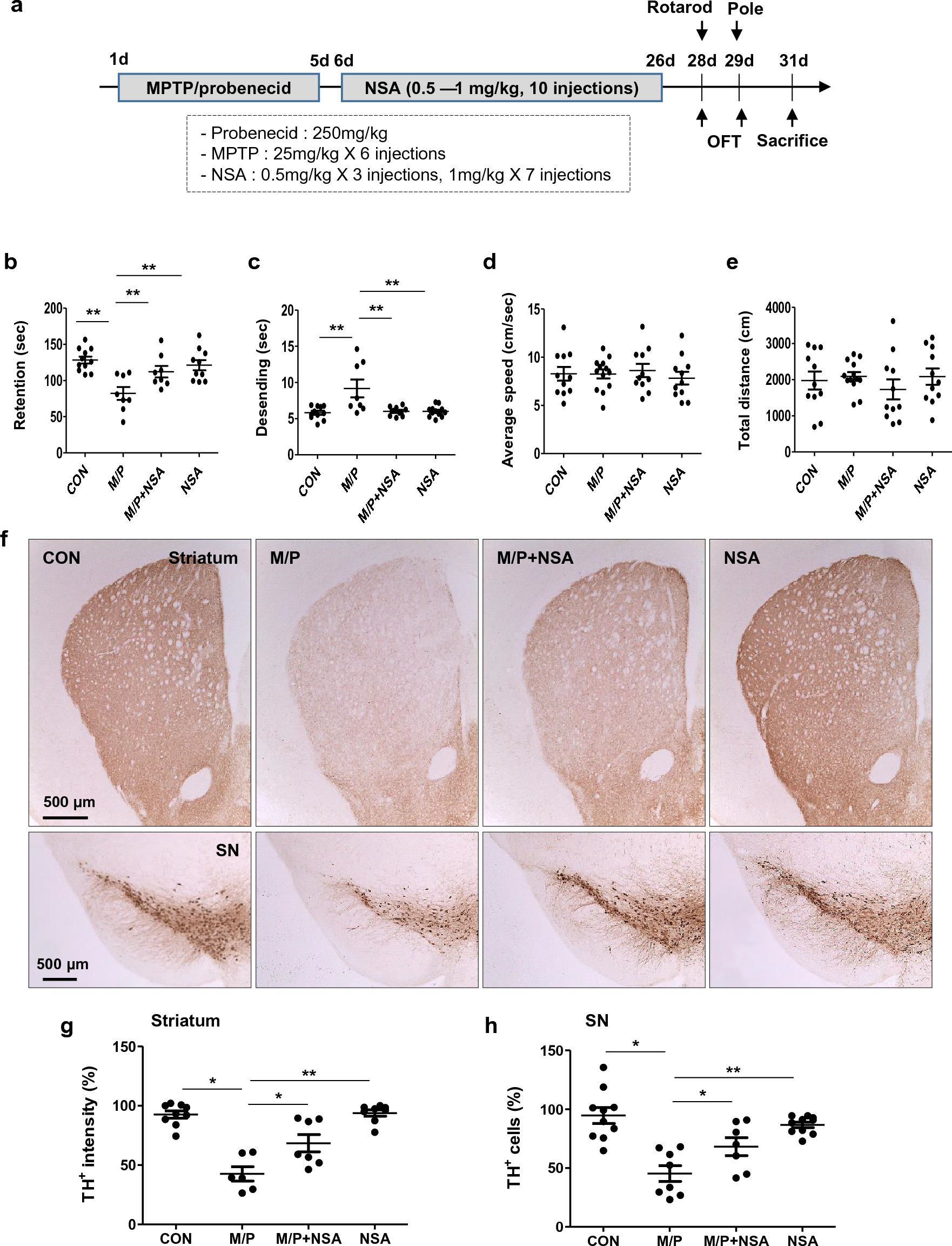The image is a detailed scientific diagram consisting of various graphs and microscopic images. It is centered on 8 close-up photos arranged in two rows, with the top row of four images being slightly larger vertically than the bottom row. The images depict an orangey material, likely some sort of tissue or cellular samples, with variations in color intensity from lighter to darker shades of pink and orange. 

Each image is labeled with abbreviations such as "CON," "M-P,” “M-P plus NSA,” and “NSA.” These labels indicate different experimental conditions or treatments, possibly involving MPTP and probonic acid, with one milligram per kilogram and ten injections noted.

Above the rows of images, there are multiple graphs and charts featuring metrics like retention, average speed, total distance, and descending seconds. The top of the diagram is marked "Figure A1D," and includes references to MPTP/probenecid treatments. Additional scatter-type graphs at the bottom are labeled "striatum" and "SN," detailing further data points.

The overall background of the diagram is light blue, contrasting with the dark pink and reddish-brown hues of the images, suggesting detailed microscopic analysis, possibly of stained tissue or bacterial samples. The graphs display quantitative data with various metrics over time, marking different days and conditions, meticulously documenting the experimental observations.